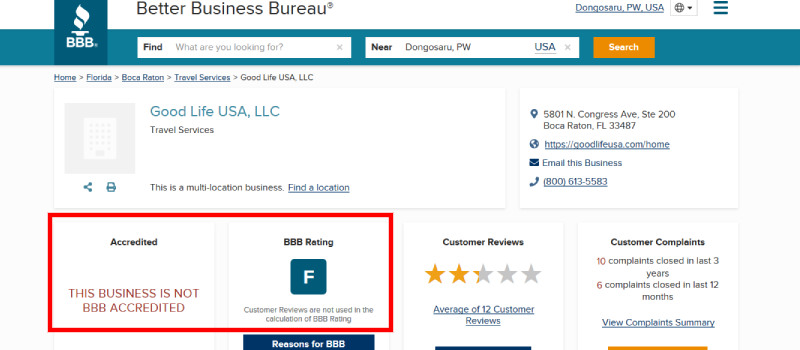This is an image of the Better Business Bureau (BBB) website. At the very top, there is a white border about an inch wide. Approximately an inch from the left edge, a dark blue square features the BBB logo: three white capital letters "BBB" beneath two white flames and a small stand.

To the right of the logo, the text "Better Business Bureau" is displayed in dark blue. Further right, an address reads "Dongasora, PW, USA." Beside this, there is an icon consisting of a small circle within a square, flanked by three blue lines.

Below that top section, an inch-wide blue border spans the width of the page. Directly beneath the "Better Business Bureau" text is a rectangular search button asking, "What are you looking for?" Next to this, there is a search tab labeled "Near," which helps locate nearby places. This tab includes an orange section with white lettering that reads "Search."

The majority of the remaining web page is white. Across the top, additional options include "Home," "Florida," "Baton Rouge," and "Travel Services" in blue text. Below these, a company name, "Good Life, USA, LLC," is displayed.

In the bottom left corner of the section, a small red rectangle reads "Accredited." Below that, the text states, "This business is not BBB accredited" in red. On the right side, a segment labeled "BBB Rating" accompanies a blue square displaying a white "F."

To the right, there is an address, a link to "Good Life, USA," an email link, and a phone number link. Beneath these, a customer review section shows a rating of a little less than two and a quarter stars. On the right side of this review section, it notes there have been ten customer complaints in the last three years and six complaints in the last twelve months.